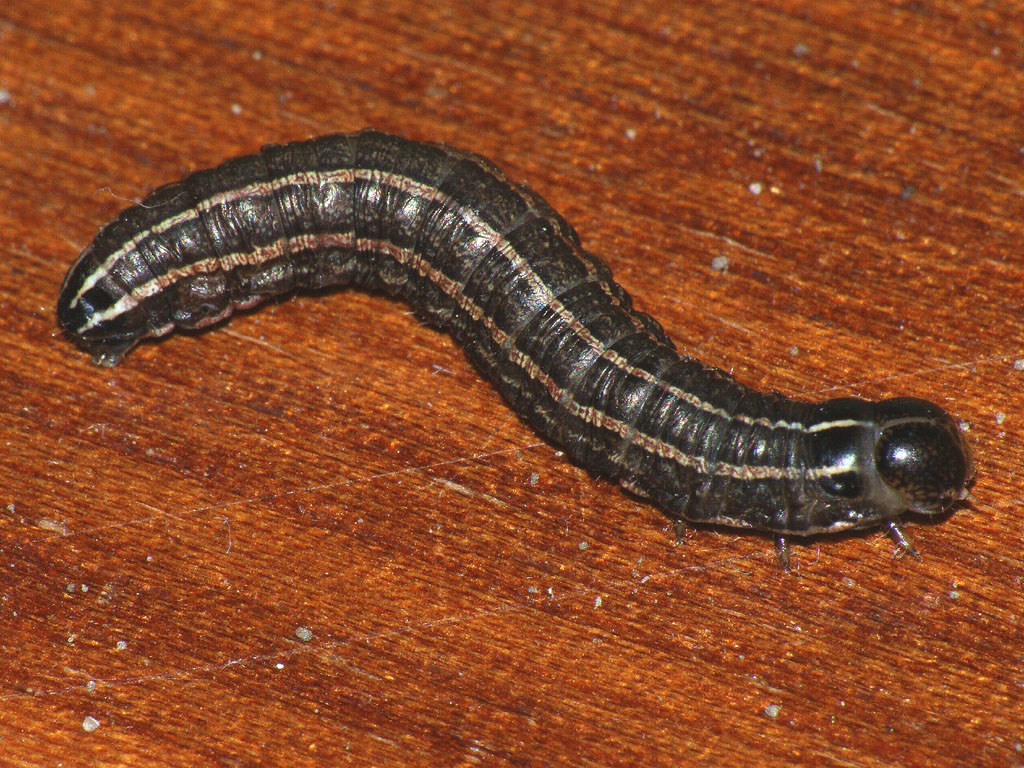The photograph is an up-close shot of a fat caterpillar on a textured brown wooden surface, which shows scratches and an orangey-brown color. The caterpillar features a long, shiny black body adorned with reflective ridges and goldish-brown stripes, including two prominent stripes running down its sides. Its numerous stubby legs are visible along its body, emphasizing its segmented structure. The caterpillar's head is dominated by two large black eyes, composed of many almost brown shapes, giving them a highly detailed appearance. The caterpillar's body is arched in a shape that can be described as a loose question mark or an S curve, with its head facing to the right while the body extends up to the upper left and then arcs back down to the middle left.